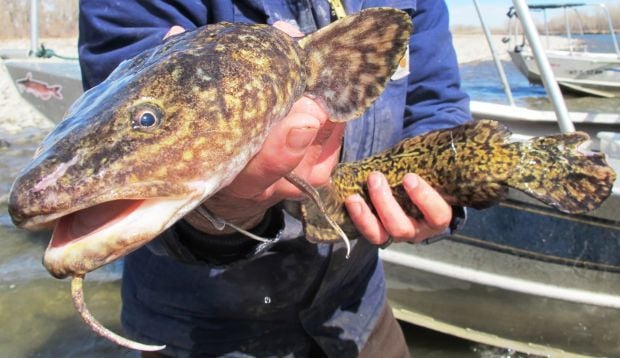In this detailed image, a man is holding a large, whiskered fish—likely a catfish—in both hands. The fish's head is in his right hand, and its elongated body, marked with green and black speckles, extends to his left hand, curving slightly. The fish's face is oriented towards the camera showing its eyeless shock and two prominent whiskers. The man, dressed in a blue jacket and black pants, has his torso and part of his leg visible, though his face is not shown. He has dirty fingernails and the fish is held firmly, with the open mouth next to the camera on the left side of the image. Behind the man, there's a white boat with a blue stripe and a catfish sticker on the bow, indicating a metallic material, and further beyond, another white boat. The background reveals a blue river flowing on the upper right and a distant shoreline, suggesting the setting is near a marina on a sunny day.